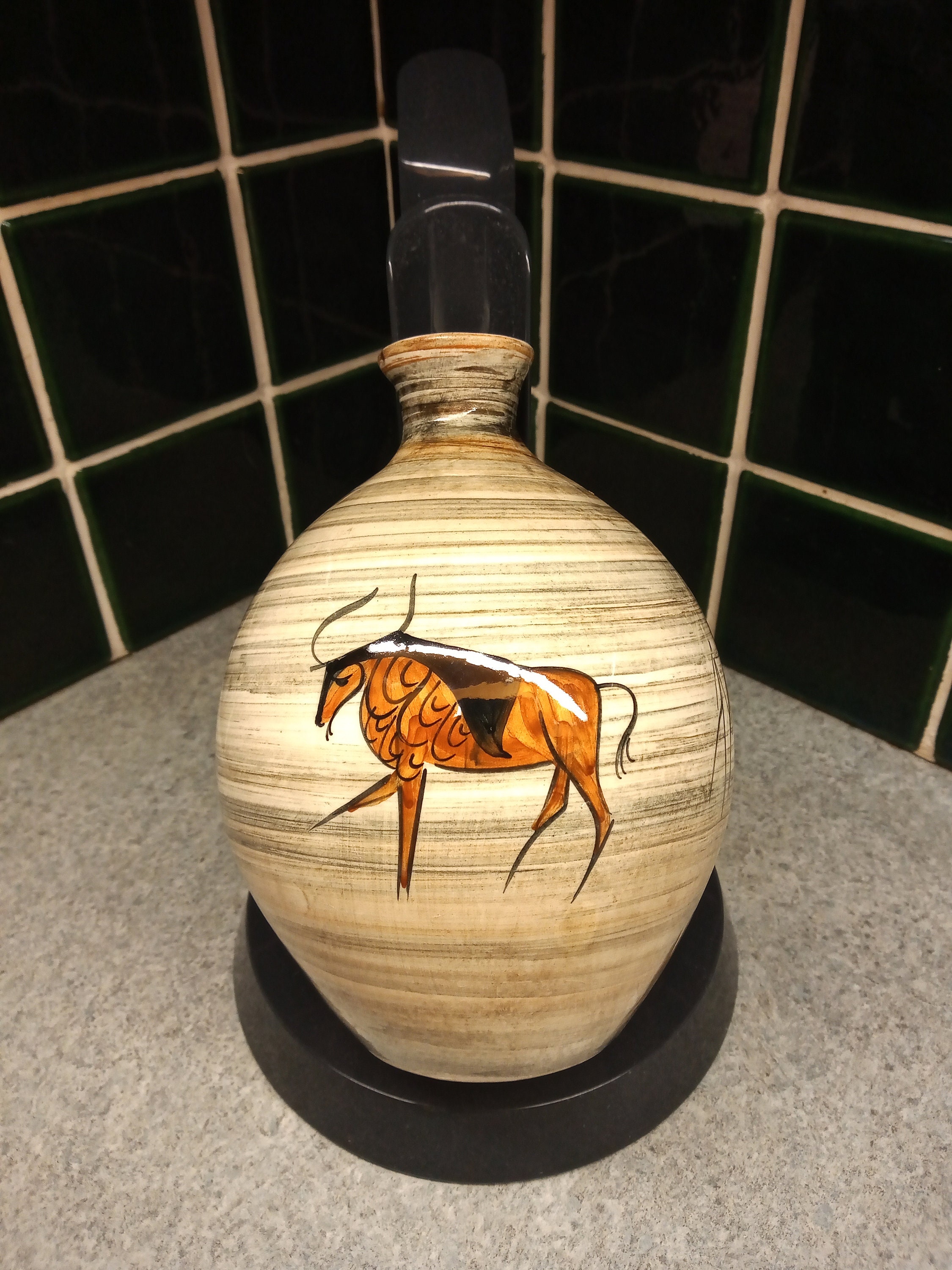The photograph showcases an ancient, bulbous vase perched on a black circular stand atop a gray marble surface. The background features two adjoining walls adorned with black tiles separated by white grout. The vase itself appears to be of significant age, with a predominantly brown, slightly tan hue and horizontal stripes of varying tan shades adorning its surface. A simplistic yet detailed depiction of a horned animal, likely an ox or long-horned antelope, is prominently displayed in the center. This creature is rendered in medium brown with a dark brown mane, narrow legs, two thin horns, a small beard, and a wispy tail. The vase has a black, glass-like top that slightly flares out, complementing the overall ancient aesthetic captured in a museum-esque setting.